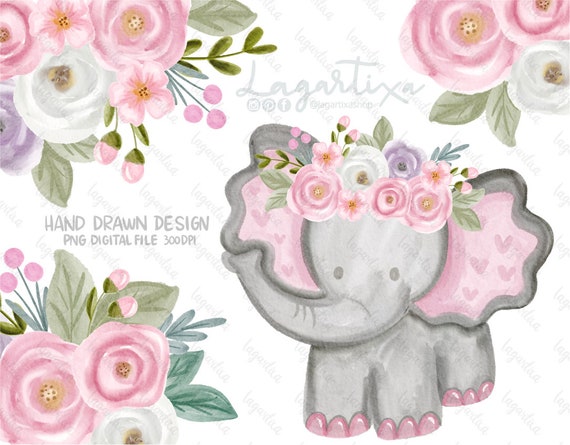The image showcases a charming hand-drawn design of a cartoon-style gray elephant with a dark gray outline, set against a white background. The elephant features pastel pink toenails and inner ears, matching the delicate floral crown adorning its head. This crown comprises pink roses, white roses, and a purple flower interspersed with green leaves. Surrounding the elephant are three similar bouquets of pastel pink roses, white flowers, and green leaves, located in the top right, top left, and lower left corners. The light gray text "Hand Drawn Design, PNG, Digital File, 300 DPI" is visible on the left side, while "Legartix" is faintly inscribed at the top, making the image suitable for a young girl's decor.